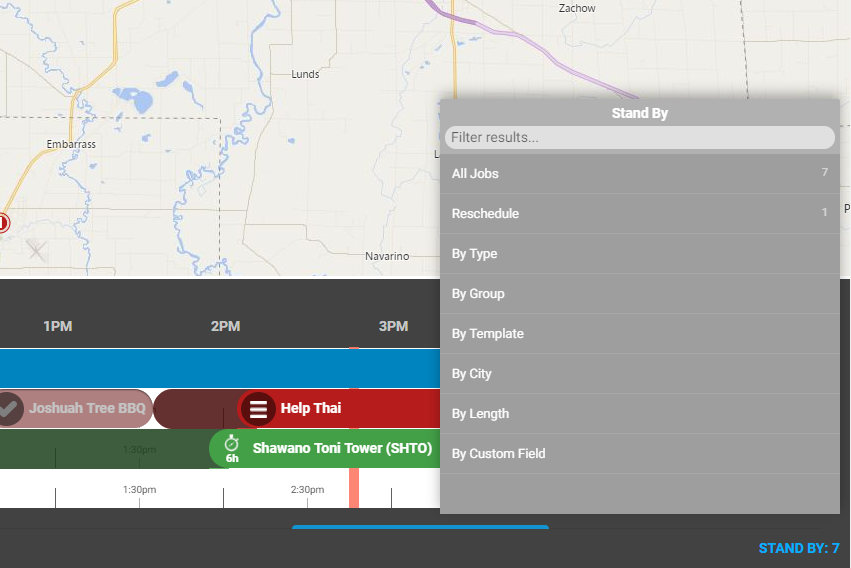This image depicts a detailed map and scheduling interface, with various elements and labels for both geographical locations and job tasks.

**Upper Portion:**
- A map is displayed prominently, with "Embarrass" labeled at the far left, indicating a specific location.
- Moving towards the center, another location is marked as "Luns."
- "Navarino" is labeled towards the bottom of the map, and "Zachow" appears towards the top-right area.
- The map includes several colored lines (yellow, purple, blue) which likely represent roads or boundaries of properties or locations.

**Right Section:**
- There is a gray rectangle labeled "Standby."
- Below this, a text box provides additional context: "Filter Results: All Jobs 7, Reschedule 1, By Type, By Group, By Template, By City, By Length, By Custom Field."

**Left Section:**
- Time markers are listed vertically from "1 PM" to "3 PM."
- A red rectangle highlights an entry labeled "Joshua Tree BBQ."
- Adjacent to this, the text "Help Tie" appears against a red background.

**Center and Lower page:**
- An image of a stopwatch is displayed, with the accompanying text "6H."
- Below this, "Shawano Tony Tower, S-H-T-O" is noted, with times "1.30 PM" and "2.30 PM" listed.
- Finally, the bottom right corner of the page indicates "Standby 7."

This caption combines geographic information with a clearly segmented scheduling interface, providing an organized overview of the map and associated tasks listed on the page.